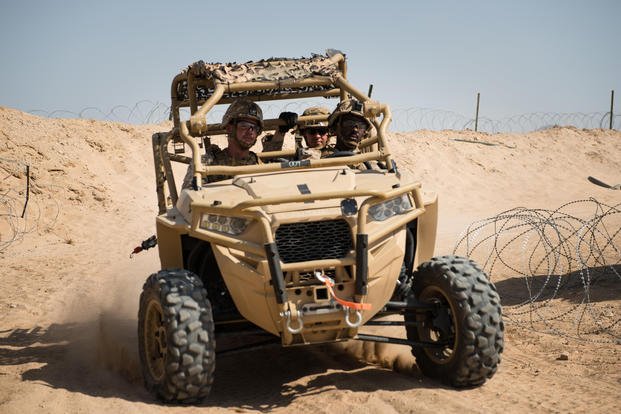In this color photograph, we see an off-road vehicle, likely a dune buggy or ATV, navigating a harsh desert terrain under a bright, heavily sunlit sky that appears gray from the intense light. The vehicle is painted a light tan and is equipped with massive black tires with substantial treads, ideal for the sandy environment. It features robust roll bars, some wrapped in desert camouflage, to protect its occupants. At the front, there are heavy-duty bars and headlights.

The vehicle, with three to four soldiers aboard, is seen moving past coils of barbed wire and stakes embedded in the sandy landscape. These soldiers are donned in full military gear, wearing camouflage helmets and goggles, with the rear soldier additionally sporting sunglasses. Surrounding the scene is a light tan expanse of desert sand, accentuated by small mounds of dirt. The sparse vegetation and presence of barbed wire suggest a war zone, underscoring the vehicle's utilitarian and resilient design for such harsh conditions.